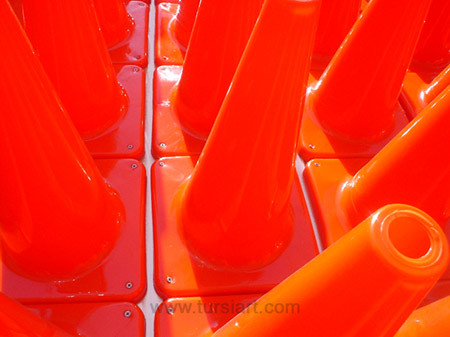This close-up photograph features approximately a dozen orange safety cones, typically used in construction zones or accident sites by services like Caltrans. The cones are arranged in three or four neat rows, with small gaps of white space between them, emphasizing their individual separation. Made of rubber, these cones are depicted from a top-down perspective, filling the entire frame of the image. Each cone is detailed with grey screws at their bases, adding to the realism of the scene. A faint watermark, www.somethingart.com, is visible at the bottom, but it is quite faded and hard to discern.